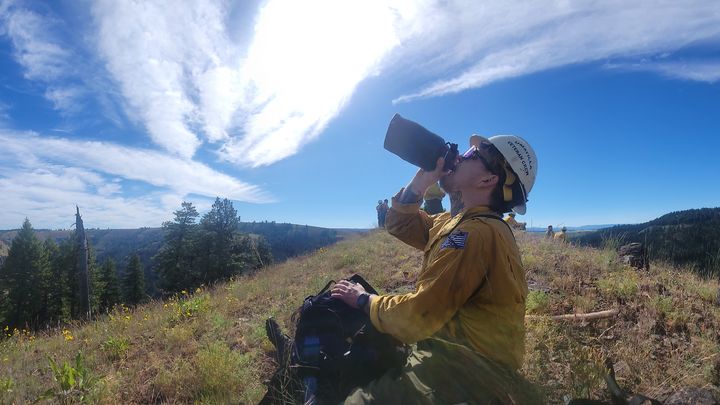This photograph captures a sunny, blue-skied day in the great wilderness, featuring a mix of natural elements and a central figure engaged in an outdoor activity. Wispy, white clouds linger in the upper left corner of the bright blue sky. The scene is set in a high-elevation, hilly area with brown-green grass and scattered yellow flowers, possibly dandelions. 

The focal point is a white male seated in the center towards the bottom of the image. He faces the left and drinks from a canteen or thermos. He dons a long-sleeved, orangish-yellow shirt, green pants, and accessorizes with a white hard hat adorned with black writing, a wristwatch, and sunglasses. Notably, he sports tattoos on both his neck and wrist. A hiking backpack rests on the ground in front of him. 

In the background, far off in the distance, are other hikers standing. Surrounding the scene, tall pine trees rise to the left, while a large tree-covered hill or mountain is visible on the right. Another tree-covered hill is faintly discernible behind the trees on the left. The overall landscape suggests a rugged, yet serene setting ideal for outdoor adventure.